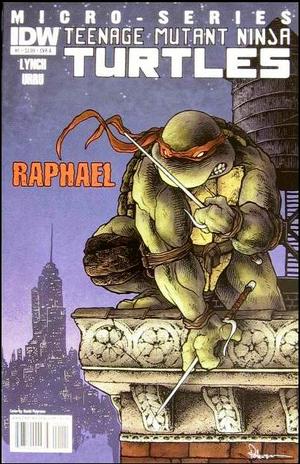This cover of the comic book from the Micro Series Teenage Mutant Ninja Turtles features Raphael, the red-masked turtle, front and center. The title "Raphael" is written in an orange hue at the top. Raphael is perched like a gargoyle on the corner of a brick building, his body hunched over as he peers down with an angry expression on his face. His iconic red mask is depicted with flowing ribbons trailing behind him in the dark blue or purplish night sky. He wields two sai; one is clenched upright in his right hand, while the other is clawed into the building's side with his left hand. Behind him, a water tower rises from the roof, and in the far distance, a tall skyscraper with its spire illuminated stands against the cityscape. Additionally, the background is tinged with purple gradients, suggesting the time might be dawn. The bottom left corner of the cover features a barcode for scanning, and the IDW logo is prominently displayed at the top left.